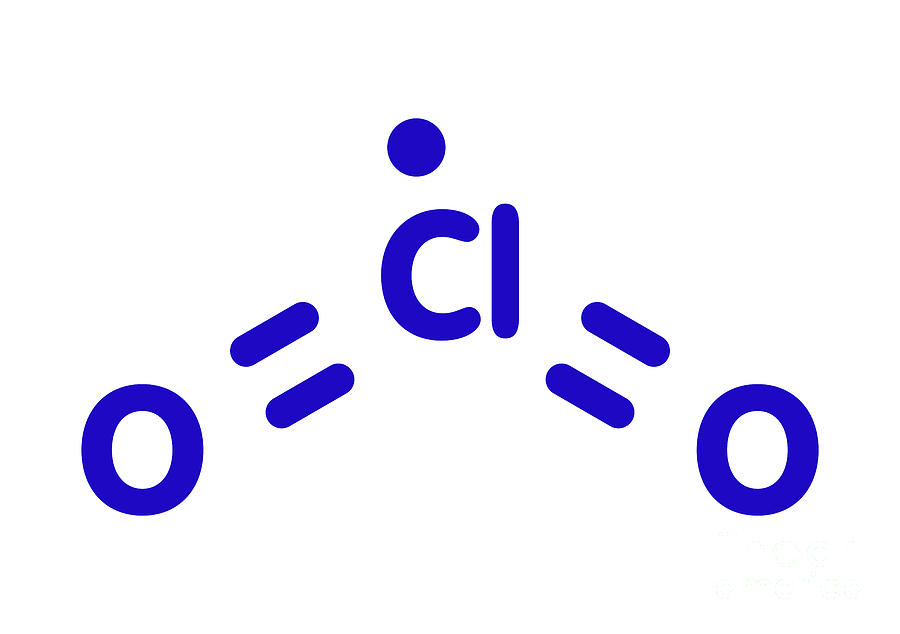The image depicts a chemical structure illustration in dark navy or royal blue text on a white background. At the left side of the image, there's an oxygen atom symbolized by the letter "O", which is connected by a double bond (depicted as two horizontal parallel lines) to a central chlorine atom denoted as "Cl". Notably, above the "C" in chlorine, there's a large blue dot, potentially indicating a special notation or charge like a chloride ion. The chemical structure continues with another double bond extending from the chlorine atom to a second oxygen atom, again symbolized by the letter "O" on the far right. The entire structure forms a linear representation of the molecule, emphasizing the connections and bonds between the atoms.